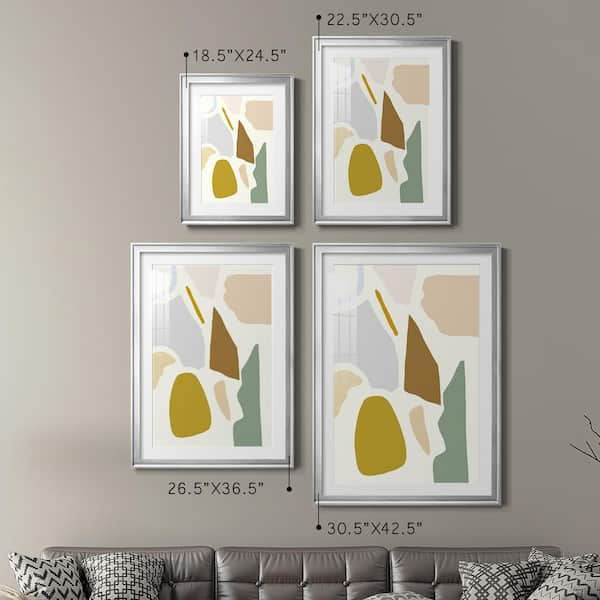The image captures a cozy yet modern living room scene with a metallic silver couch adorned with patterned black and white pillows. The backdrop is a plain, light gray-beige wall, which serves as a canvas for a striking arrangement of four silver-framed, abstract art prints. The frames are meticulously organized, with the smallest on the top left, measuring 18.5 by 24.5 inches, and to its right, a slightly larger one at 22.5 by 30.5 inches. Below these, on the bottom left, there is a frame sized at 26.5 by 36.5 inches, and the largest frame on the bottom right, measuring 30.5 by 42.5 inches. Each print within the frames appears to be a variant of a creative abstract design, adding a cohesive yet dynamic element to the sophisticated and serene ambiance of the room.